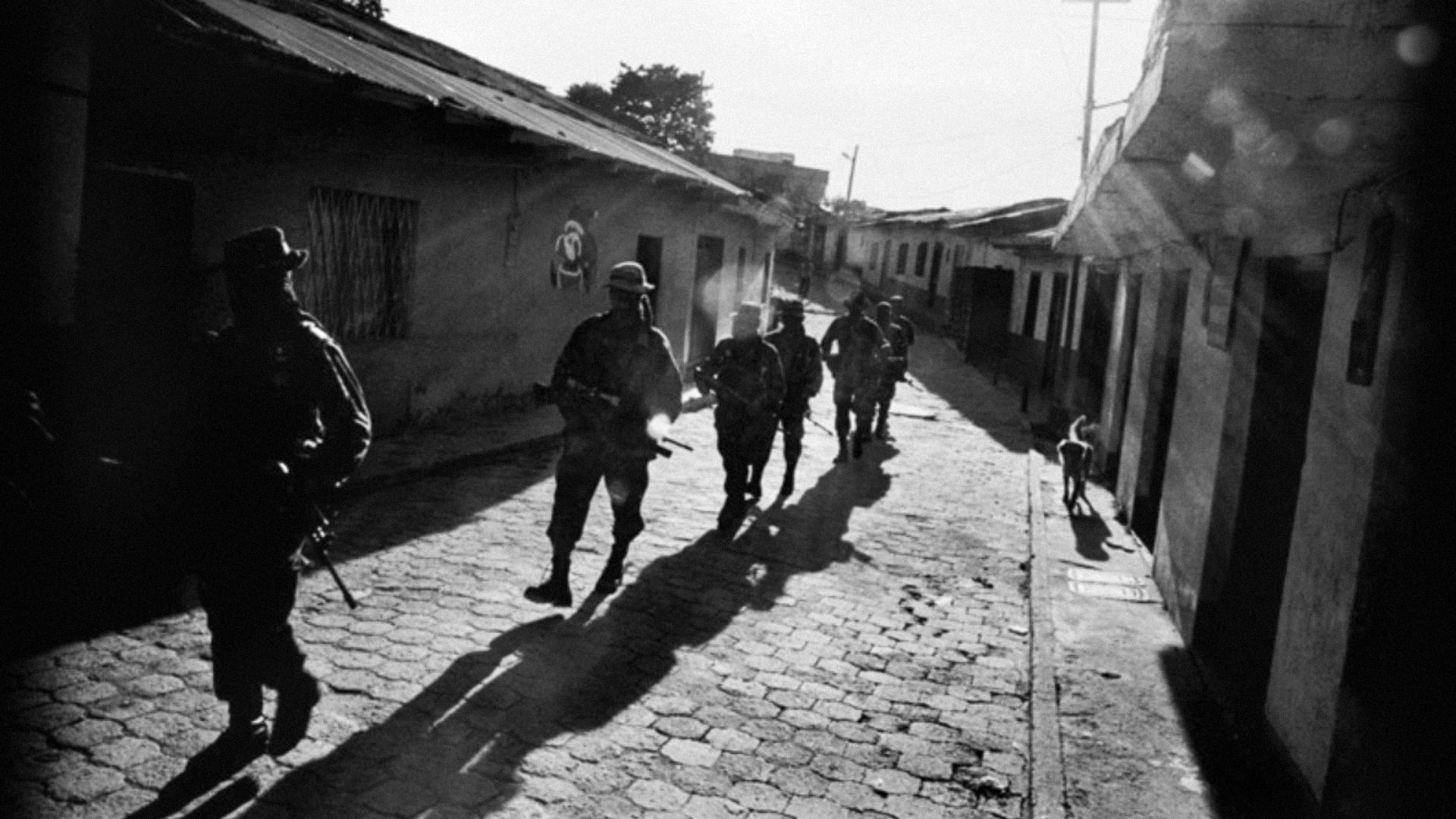In this striking black and white photograph, a group of seven or eight armed soldiers march in single file along a narrow, curving cobblestone street, their backs to the camera. The street is flanked by modest buildings, representative of a small, impoverished town that evokes a sense of vulnerability amidst the backdrop of potential conflict, possibly somewhere in Latin America such as Guatemala or Mexico. Despite the urban setting, there is an eerie calm, with no sign of an active engagement. The soldiers, donned in camouflage and light caps, grip their rifles as they proceed, seemingly in search of something or someone. A lone dog stands on what could pass for a sidewalk, contributing to the quiet tension of the scene. The photograph, taken during daylight, features strong light that leaves the men dramatically backlit against a bright, white sky, enhancing the contrast and the somber mood of the image.